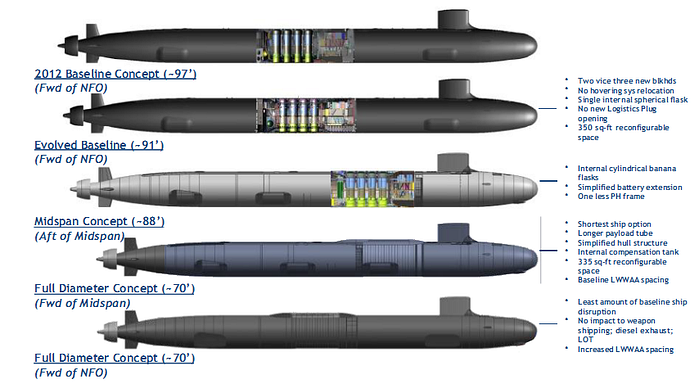The image showcases a detailed graphic of five cylindrical objects reminiscent of submarines, torpedoes, or potentially missiles, stacked vertically in a sequential arrangement against a white background. The top cylinder is black and labeled "2012 Baseline Concept." Below it, a second black cylinder is marked "Evolved Baseline, forward of NFO-91." The third object, silver, is designated "Mid-Span Concept-88, AFT of Mid-Span." The fourth, dark gray transitioning to lighter gray, bears the label "Full-Diameter Concept-70, forward of Mid-Span." The final cylinder, solid black, is titled "Full-Diameter Concept-70, forward of NFO." Alongside these objects, a bullet list enumerates various technical aspects and specifications for each concept, such as "Single internal spherical flask," "Minimum relocation," and configurations optimizing for factors like logistic simplicity and payload extension. The comprehensive layout suggests the evaluation of different design concepts within a specific engineering context.